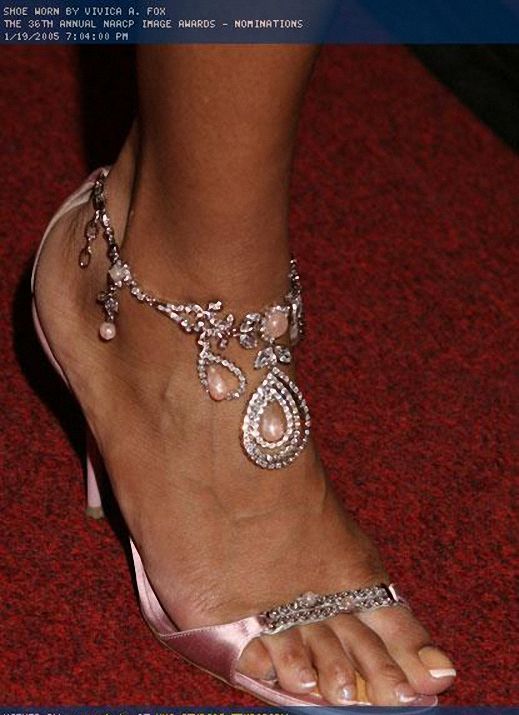The image features a close-up of a woman's right foot adorned with elegant jewelry and showcasing a meticulous pedicure. She wears a striking pink, rose gold-colored heel that wraps around her heel and extends to the toe. Across her toes lies a jewel-encrusted strap, shimmering with intricate details, while an opulent ankle strap also adorned with jewels wraps around her ankle. This strap features teardrop-shaped pendants, each set with what seems to be pink pearls and possibly rose quartz, hanging gracefully towards the center of her foot. Her toes are polished with a pristine white nail polish, set against the luxurious background of a red carpet. The top of the image features a black band with white text, indicating, "Shoe worn by Vivica A. Fox. The 36th Annual NAACP Image Awards nominations, 1-19-2005, 7:04 p.m." The overall scene captures a blend of glamor and sophistication, highlighting the detailed adornments of the jewelry and the elegance of the manicured foot.